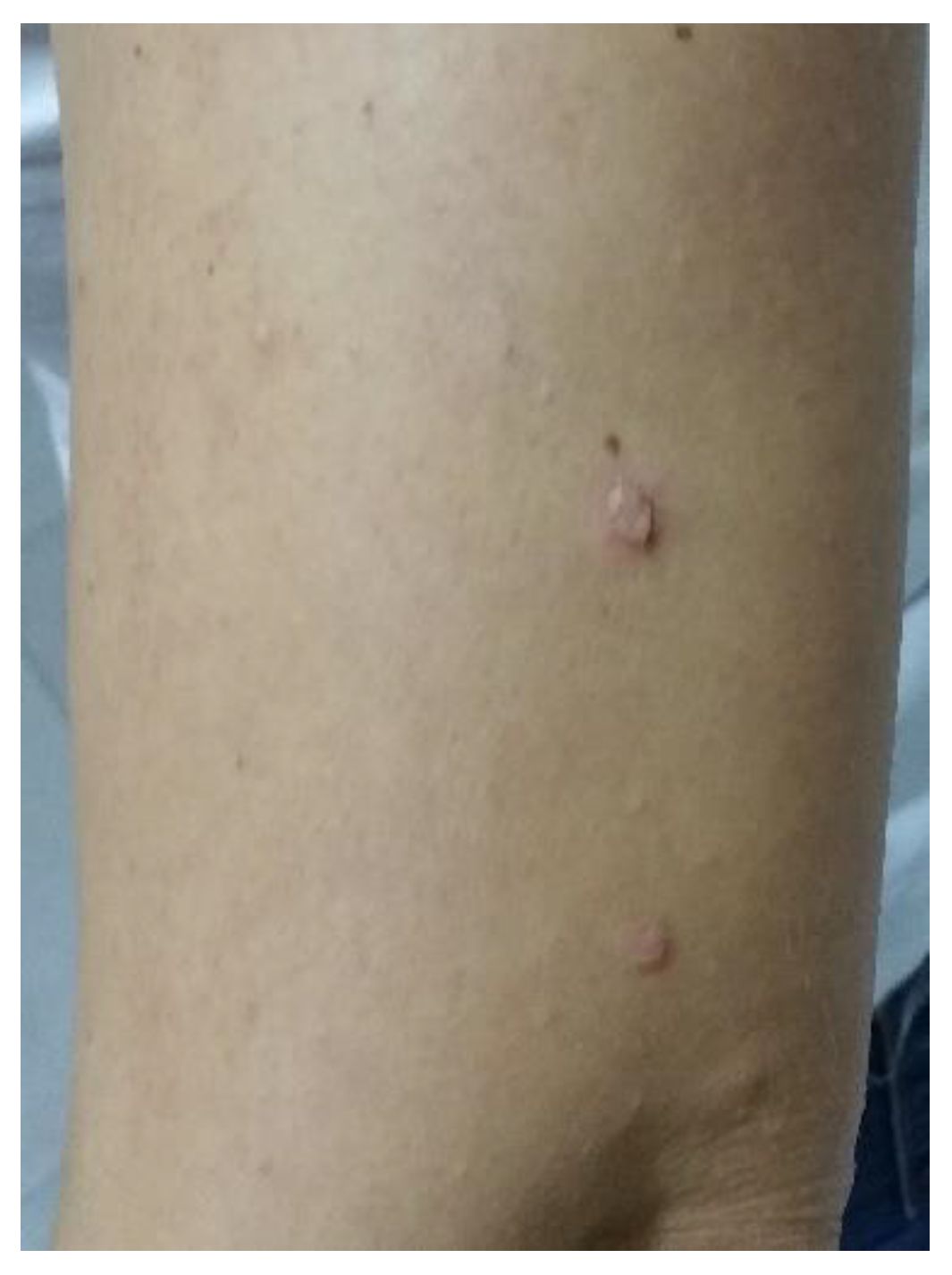The photograph, captured in portrait orientation, focuses on a person's arm, extending from just above the elbow to below the shoulder, with a light brown skin texture. The background reveals the individual is dressed in a white t-shirt and jeans. The image zooms in closely on the arm, emphasizing two red bumps on the right side. The larger bump, situated between the elbow and shoulder, is slightly raised with surrounding redness, while the smaller bump near the elbow also shows evidence of skin irritation. Additional small raised areas are visible in the bottom right corner of the frame. The style of the photograph is realistic, depicting what appears to be some sort of bug bites or minor skin infections.